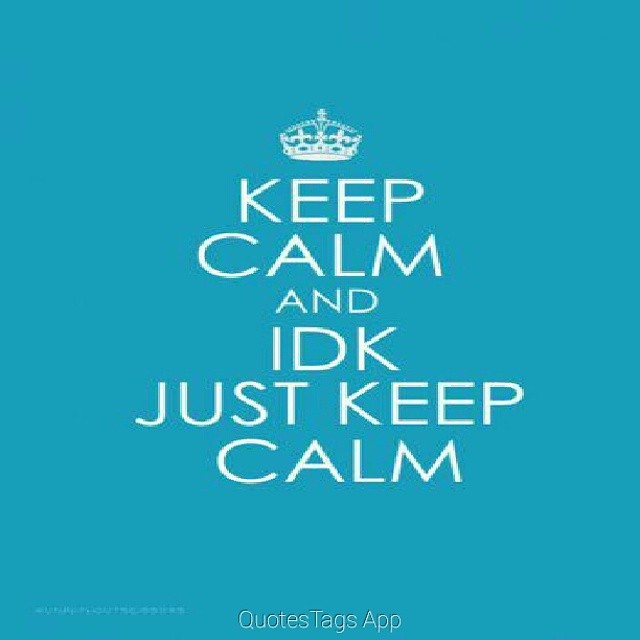The image is a square-format graphic design with a deep aqua or light turquoise background. Centered in the middle in all-white capital letters is a parody of the classic "Keep Calm and Carry On" message, adapted to read: "KEEP CALM AND IDK, JUST KEEP CALM," where "IDK" stands for "I Don't Know." Above the text is a line art illustration of a crown, also in white, maintaining the traditional format of the original phrase. At the bottom center, in light white lettering with a black border, it reads: "Quotes, Tags, App." The overall style integrates illustration and typography to create a meme-like image often shared on social media platforms like Pinterest.